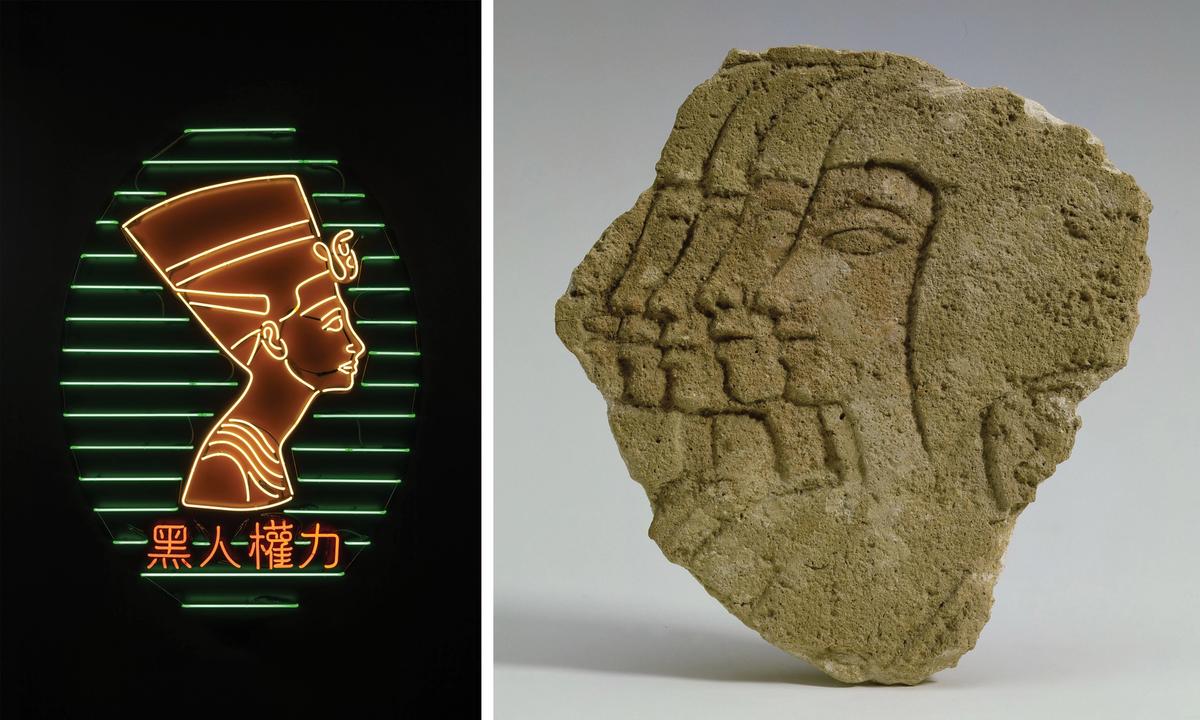The image comprises two side-by-side photographs, each featuring Egyptian themes. The photograph on the left depicts a neon sign with a black background. This sign portrays a profile of what appears to be Nefertiti, facing to the right. The profile is rendered in white neon light, highlighting the facial features and a tall headdress, complete with an asp at the front. The headdress has horizontal greenish-white neon stripes. Below this bust are four red neon Japanese characters. The figure is outlined in vibrant neon lights, set against a dark backdrop, giving it an illuminated, contemporary artistic appearance.

To the right is a photograph of an ancient Egyptian stone carving, displayed as a museum piece. The irregular chunk of stone features the profiles of four faces, one behind the other, all facing left. The first profile has the distinctive 'cat-eye' style typical of Egyptian art, and could represent either a man or a woman. The detailed carving on the stone is highlighted by a white background and excellent lighting, which accentuates the meticulous craftsmanship of the ancient artisans.